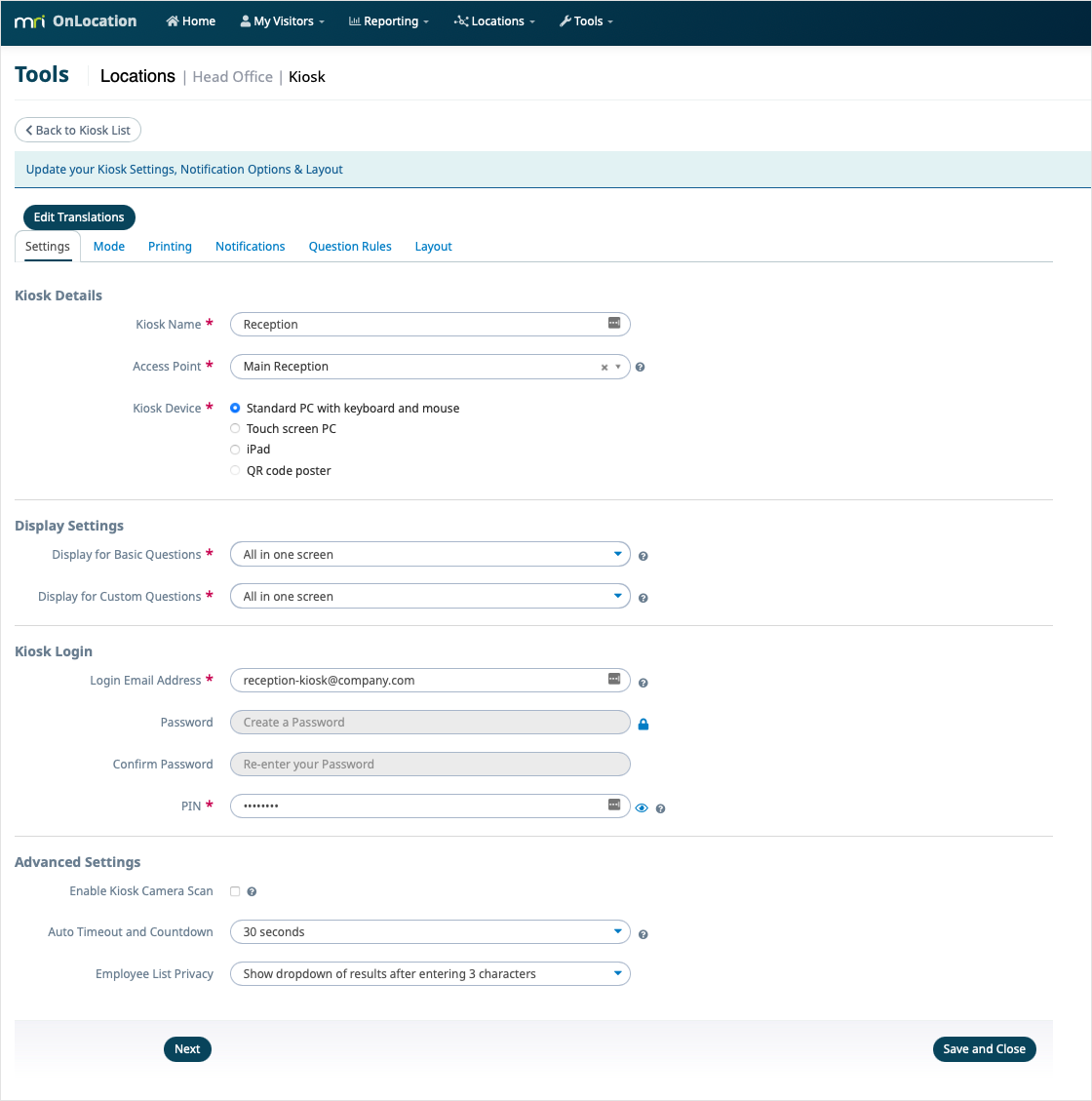The image depicts a user interface of a webpage with a prominent blue banner at the top. On the left side of this banner, "MRI" is written in white letters, followed by the text "On Location." This banner features several clickable tabs, each accompanied by an icon representing their function: a white house icon for "Home," a minimalist person for "My Visitors," a bar chart for "Reporting," a location pin for "Locations," and a wrench for "Tools."

Beneath the blue banner is a white banner containing additional tabs labeled "Locations," "Head Office," and "Kiosk." Highlighted next to these tabs is the word "Tools," indicating the current page being viewed. Just below this white banner is a tab labeled "Back to Kiosk List," complete with a backward-pointing arrow suggesting navigation to a previous page.

Further down, the page is organized into several sections with tabs labeled "Settings," "Mode," "Printing," "Notifications," "Questions," "Rules," and "Layout." All of these labels are in blue font against a clean white background, providing a clear and organized interface.